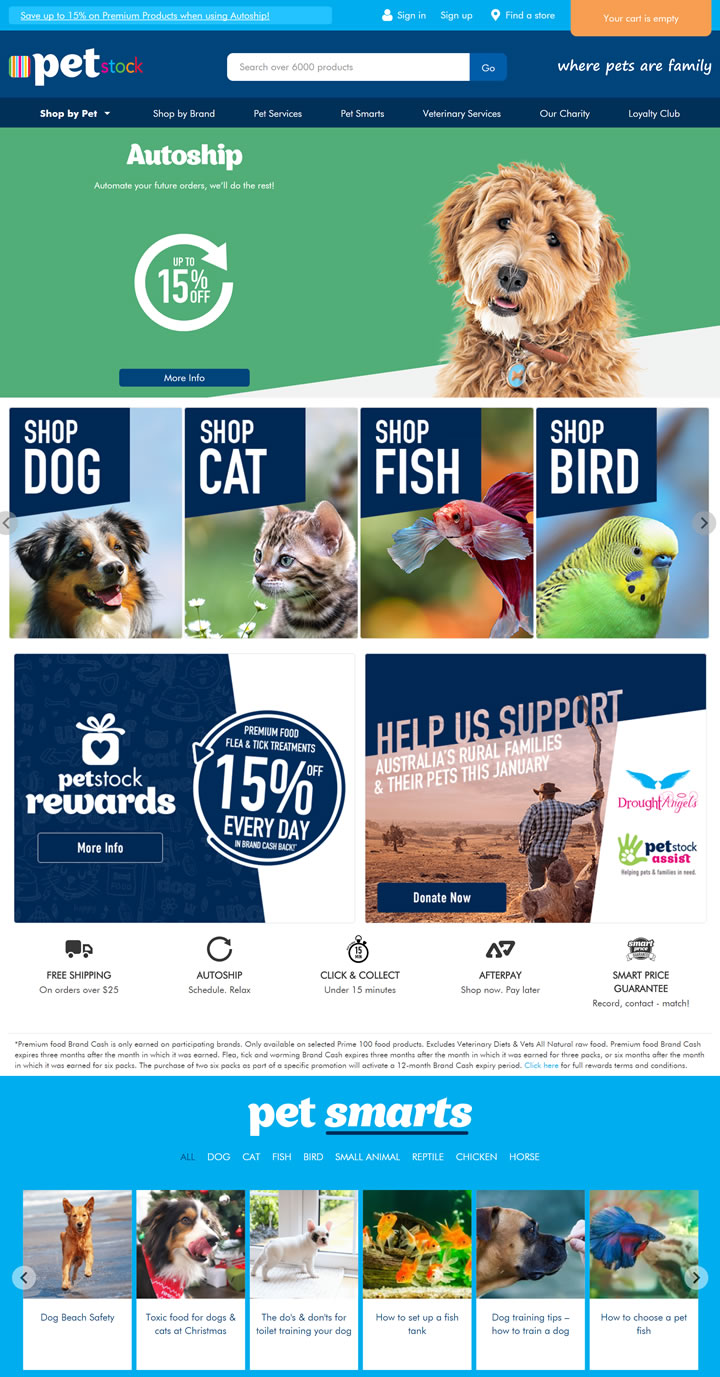This screenshot displays an online pet store's homepage featuring a variety of pet-related products and services for dogs, cats, fish, birds, and more. 

At the top left corner, the store's logo reads "Pet Stock" with "Pet" in white and "Stock" in a vibrant rainbow-colored font. Directly below the logo, there's a search bar for easy navigation. On the right, a welcoming tagline "Where Pets Are Family" is displayed. The navigation bar includes various links such as pet brand, pet services, and other essentials.

Prominently featured on the right side is an image of a brown dog gazing at the camera with a sweet and slightly sad expression. To the left, a green banner announces an auto-ship service with discounts up to 50%, accompanied by a blue "More Info" button. Below this banner, four sections labeled "Shop Dog," "Shop Cat," "Shop Fish," and "Shop Bird" are each illustrated with a corresponding animal photo. These sections use a white font on a dark blue background, inviting users to browse specific categories.

Further down, a promotional banner for "Pet Stock Rewards" offers daily 50% off rewards with a link to learn more. Another sidebar highlights a fundraising initiative: "Help Us Support Australia's Rural Families and Their Pets This January," featuring a donation button and an image of a man looking out at a desert landscape. Adjacent ads support various causes.

Near the bottom, information about shipping options, auto-ship, click-and-collect services, and other utilities are provided alongside relevant icons. The footer showcases "Pet Smarts" on a blue background, decorated with images and brief descriptions of six different animals and fish, arranged from left to right.